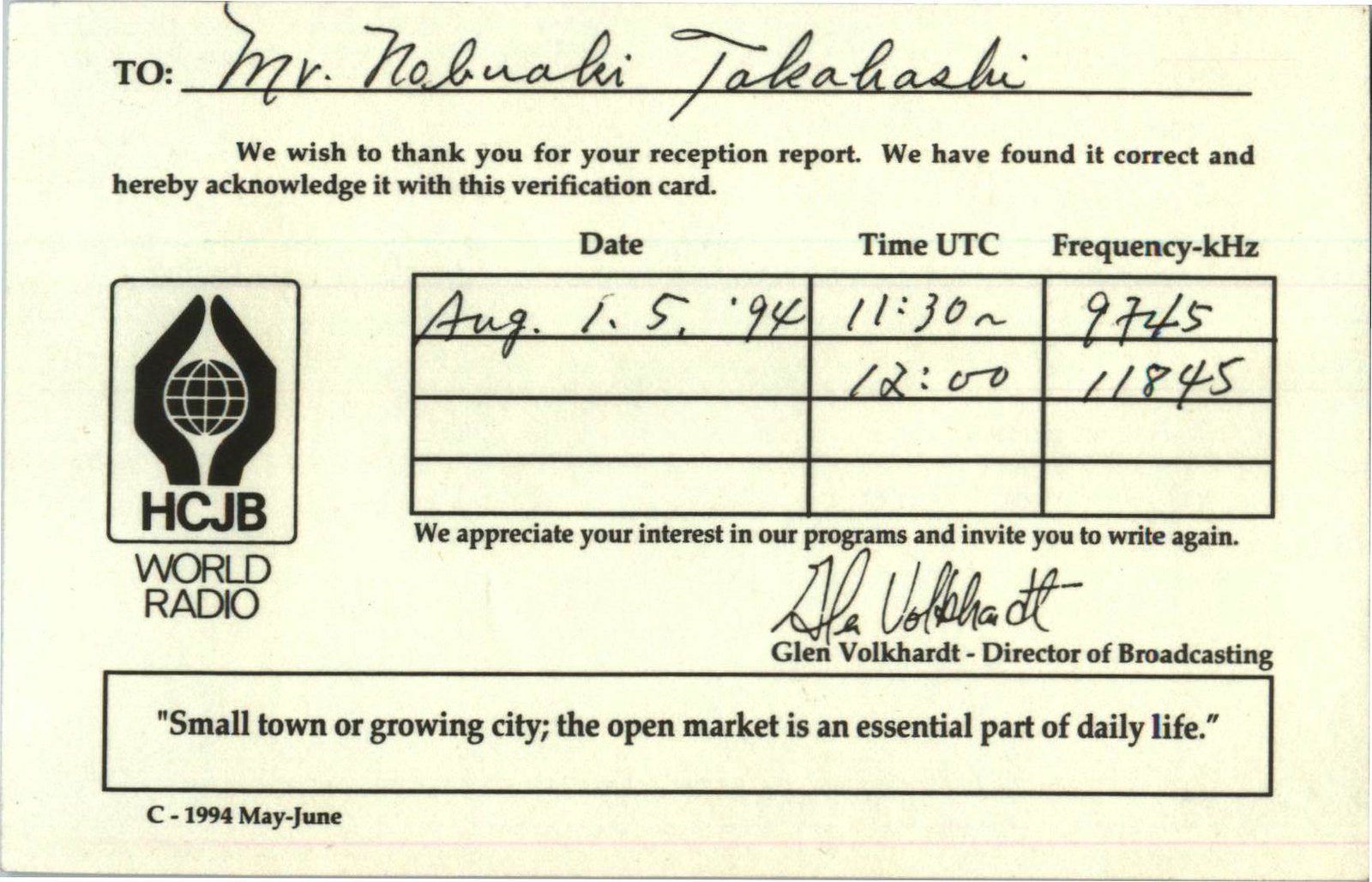The image shows a verification card from HCJB World Radio addressed to Mr. Nobuyuki Takahashi. The card, dated August 15, 1994, acknowledges his reception report for the frequencies 9745 and 11845 kHz, received between 11:30 and 12:00. It features a logo depicting hands holding a globe. The card expresses gratitude for Mr. Takahashi's interest in their programs and invites him to write again, emphasizing the value of audience interaction in shortwave radio broadcasting. At the bottom, there's a quote: "Small town or growing city, the open market is an essential part of daily life." The card is signed by Glenn Volkart, Director of Broadcasting.